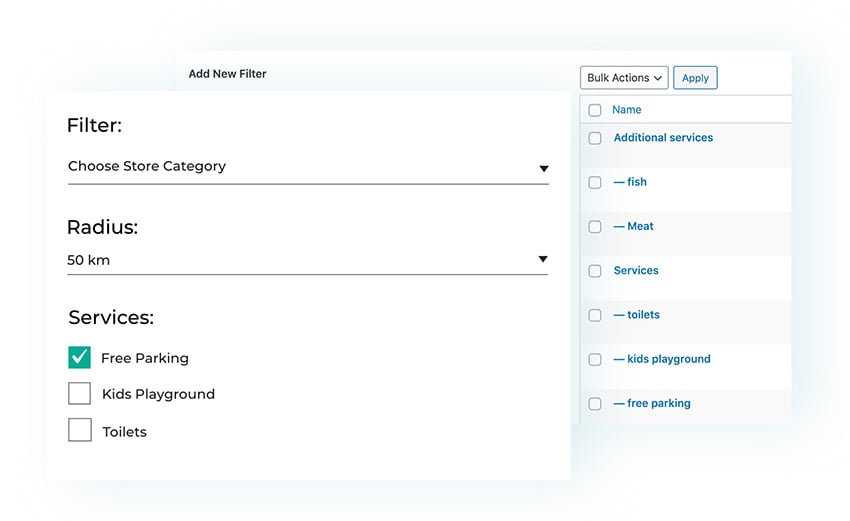The image depicts an interface for adding a new filter with various options and criteria for selecting preferred locations. At the top, there is a heading labeled "Add New Filter." Beneath this, there are fields for "Filter," "Choose Store Category," and another labeled "Radius," which is preset to 50 kilometers (KM). The interface also includes a section for selecting services, featuring options such as "Free Parking," "Kids Playground," and "Toilets," with "Free Parking" already checkmarked.

Towards the right side of the image, there is a "Bulk Actions" menu with a drop-down and an "Apply" button. Below this, there is a list of additional services each accompanied by a checkbox: "Name," "Additional Services," "Fish," "Meat," "See Services," "Toilets," "Kids Playground," and "Free Parking." Users can check any of these options to filter their search results more precisely. The interface appears to be designed to help users find locations like restaurants or parks that offer specific amenities for convenience and requirements.